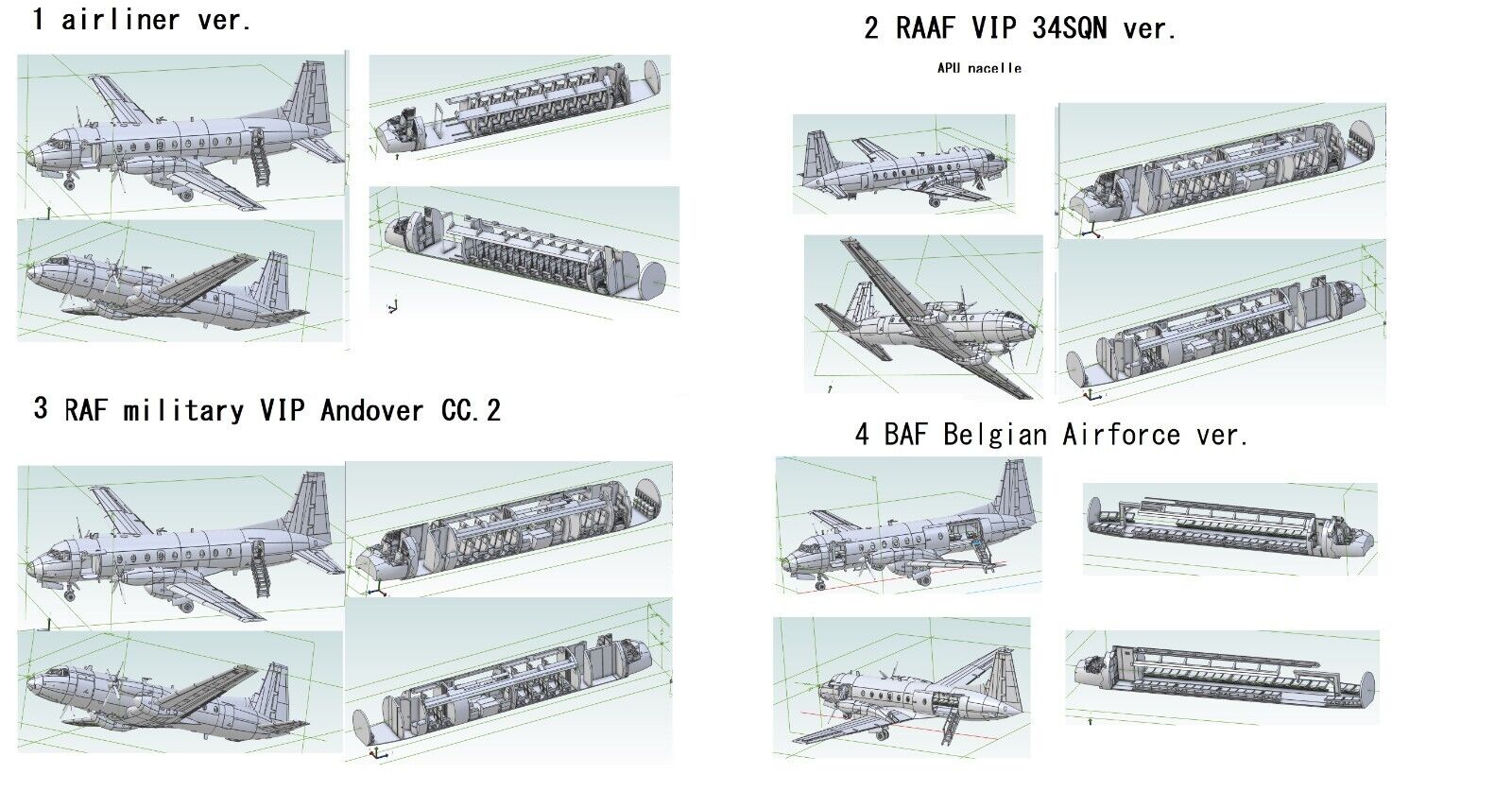The image showcases four detailed architectural designs of aircraft, each from different countries. These blueprints are meticulously rendered in gray and light blue tones and are arranged in four distinct sections. The top-left section illustrates the "Airliner Version" (VER), featuring comprehensive 3D diagrams of the aircraft, including top views, wings, and interior layouts without the exterior shell. Adjacent to this, the top-right section is labeled "RAAF VIP 34 SQN Version" and similarly presents the aircraft from multiple perspectives, highlighting both external and internal configurations. The bottom-left section, marked "RAF Military VIP Andover," continues this detailed examination, depicting the aircraft from various angles and interior schematics. Finally, the bottom-right section shows the "BAF Belgian Air Force Version," maintaining the same meticulous detail with multiple views and interior insights. Above each section, black lettering identifies each design, creating a cohesive and informative visual representation of these international aircraft versions.